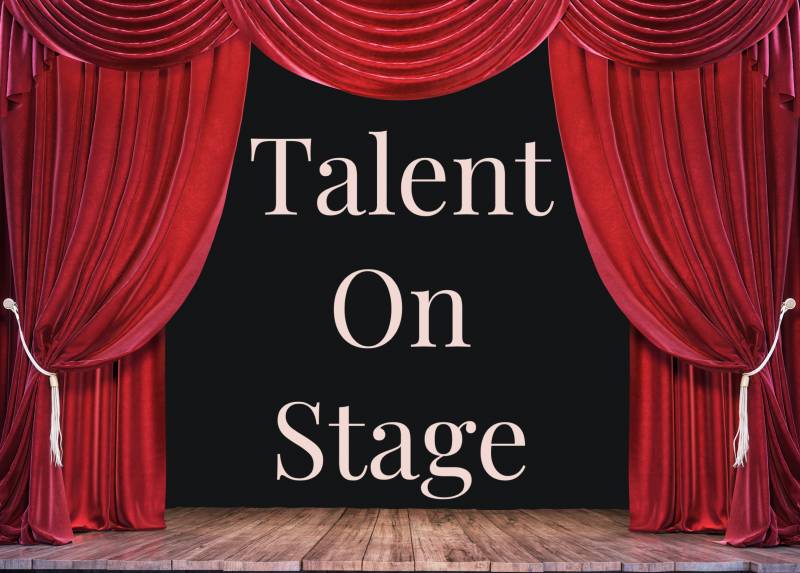The image portrays a classic theatrical stage scene. Dominating the space are rich, red curtains, which are tied up with off-white ropes, revealing a black backdrop in the center. The curtains, adorned with a stringy texture, cascade elegantly from top to bottom. The focal point of the backdrop is the large, prominent text reading "Talent on Stage" in an off-white, light pinkish hue. Below the dramatic curtains lies a lustrous wooden floor, exhibiting varied brown tones and a glossy finish, possibly coated with epoxy. This scene is viewed from the audience's perspective, showcasing the anticipation and splendor of an upcoming performance.